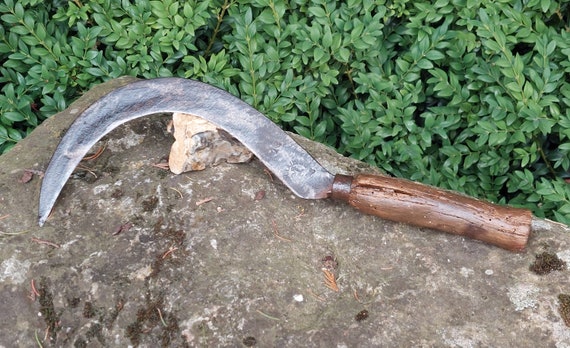This close-up photograph showcases a weathered sickle positioned on a rock. The sickle, with its silver, hooked, and visibly worn blade, lies to the left, while its medium-toned brown wooden handle, showing signs of wear, extends to the right. Between the handle and the blade is a small, darker brown section. The primary rock, which appears as a grayish slab with lighter and darker splotches, occupies much of the lower half of the landscape-oriented image. A smaller, off-white rock with gray and brown marbling underlies the sickle, elevating it slightly for emphasis. The backdrop consists of lush green bush foliage that fills the top third of the image, contrasting the sickle's metallic and wooden elements. The photograph is devoid of any other objects or individuals, drawing focus solely to the sickle and its supporting surfaces.